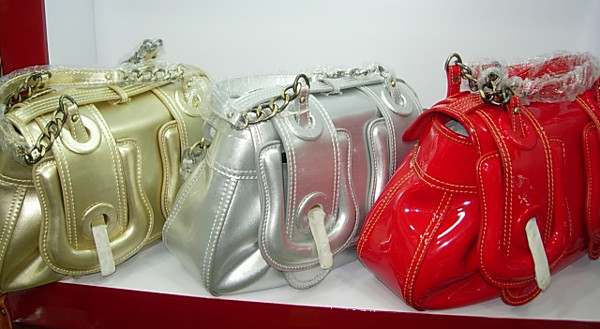This realistic photograph showcases three stylish and fashionable handbags displayed within a white alcove set against a red wall. The image is bright and well-lit, suggesting it was taken indoors, possibly inside a store. The handbags, positioned at an angle on a white platform within the alcove, share an identical design with shiny, reflective surfaces and metal chain handles. Starting from the left, the handbags are gold, silver, and red, respectively. The consistent style and positioning in the minimalist setting highlight their sleek, pleather-like material and modern aesthetic. The scene is free from text, allowing the focus to remain solely on the vibrant and chic handbags.